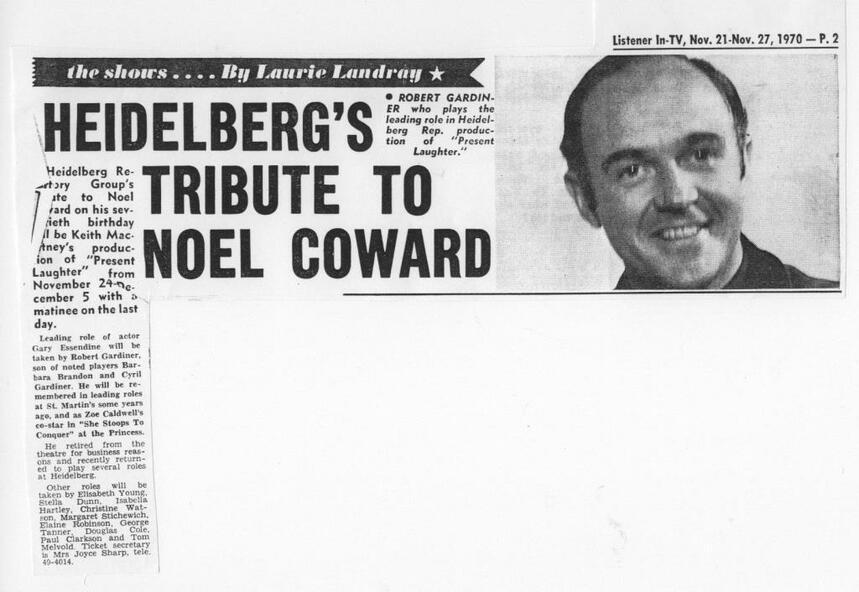This detailed newspaper clipping from November 21st to November 27th, 1970, features a black-and-white article about a tribute to the renowned playwright Noel Coward on his 70th birthday. The article is titled “The Showers” by Laurie Landry and includes an image of a smiling, middle-aged to elderly man, likely in his late 60s or early 70s, with a receding hairline and wearing a black shirt. His teeth are visible, adding to his happy demeanor. The piece highlights Heidelberg's tribute to Noel Coward, discussing productions such as "Present Laughter" featuring Robert Gardiner in the leading role of Gary Essedine, with supporting performances by other actors like Elizabeth Young. The right side of the clipping shows the gentleman's photograph, while the left side provides details about the tribute and the involved cast.